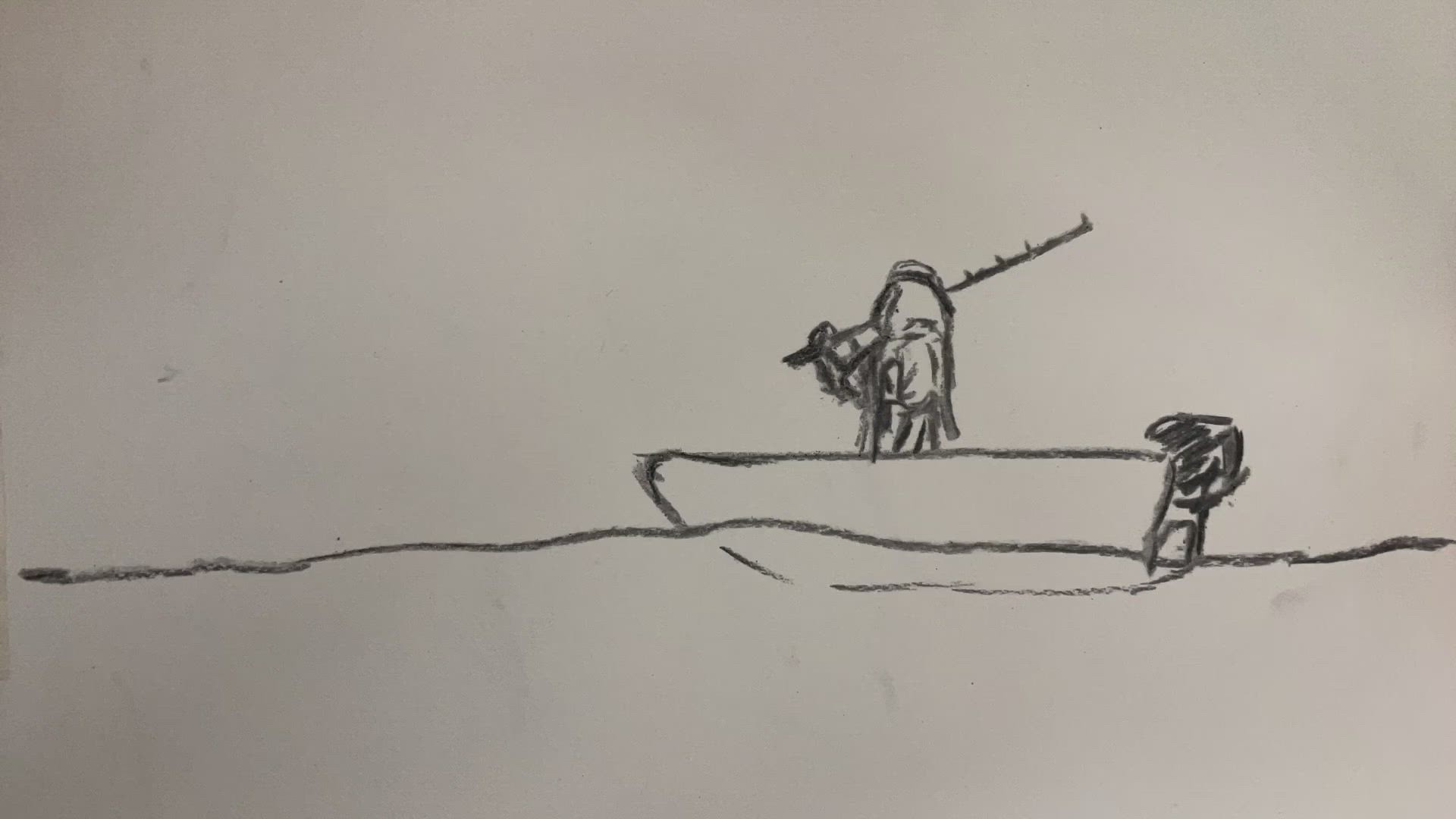This hand-drawn artwork captures a figure in a small boat, rendered on a paper-like surface. The drawing, likely created with charcoal, black watercolor, or black marker, exhibits an impressionistic style and possesses a two-dimensional quality. 

The composition is wider than it is tall, with a wavy line stretching horizontally from left to right about two-thirds to three-quarters down the paper, representing the water's surface. The boat, positioned slightly off-center to the right, points towards the left. Its size suggests it is a rowboat, though a feature at the back hints at the possibility of a motor. 

A figure, seen in side profile, occupies the boat. This person, possibly a man, holds what appears to be either a gun or a fishing pole over their right shoulder. The figure is adorned in flowing robes and wears a head covering that resembles a turban or hood, adding an air of mystique to the scene.